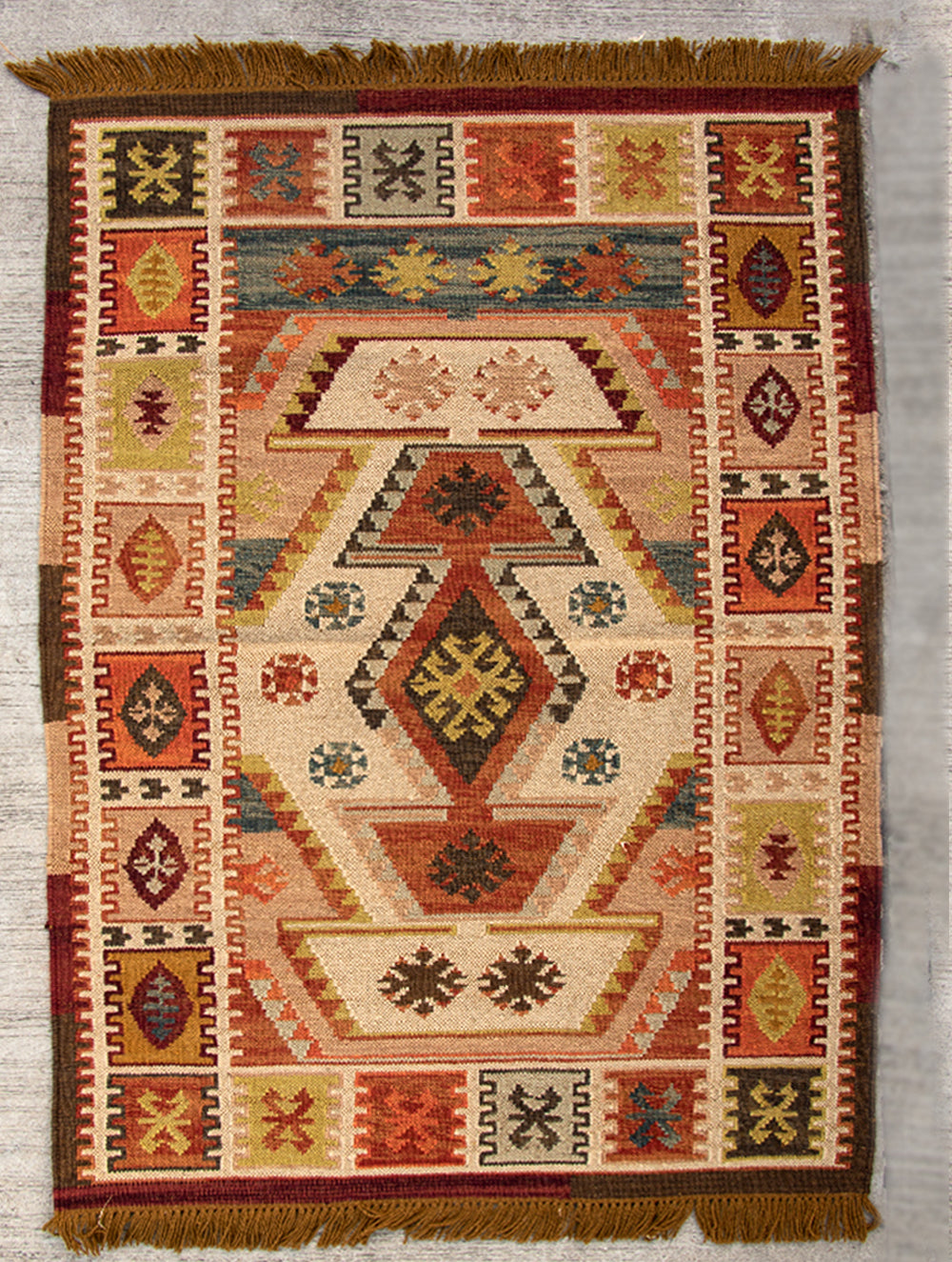This image depicts a decorative throw rug with an array of earthy tones, including oranges, browns, light greens, reds, yellows, and whites. The rug is elaborately patterned with a border of alternating black and white stripes. Within this border, the rug is divided into squares, each surrounded by designs reminiscent of tire or train tracks. The interior of each square features intricate patterns, including geometric shapes, triangles, fractal motifs, and floral prints. Notably, the center of the rug showcases red and yellow shapes resembling stars or possibly fish. Additional design elements include six circles—two in red and orange and four in green and yellow—and various geometric patterns like diamonds, triangles, and X-shaped designs. The rug also has gold-colored tassels, or frills, on both ends, adding to its southwest-inspired aesthetic. It lies on a gray floor, enhancing the visibility of its subdued but richly varied color palette.